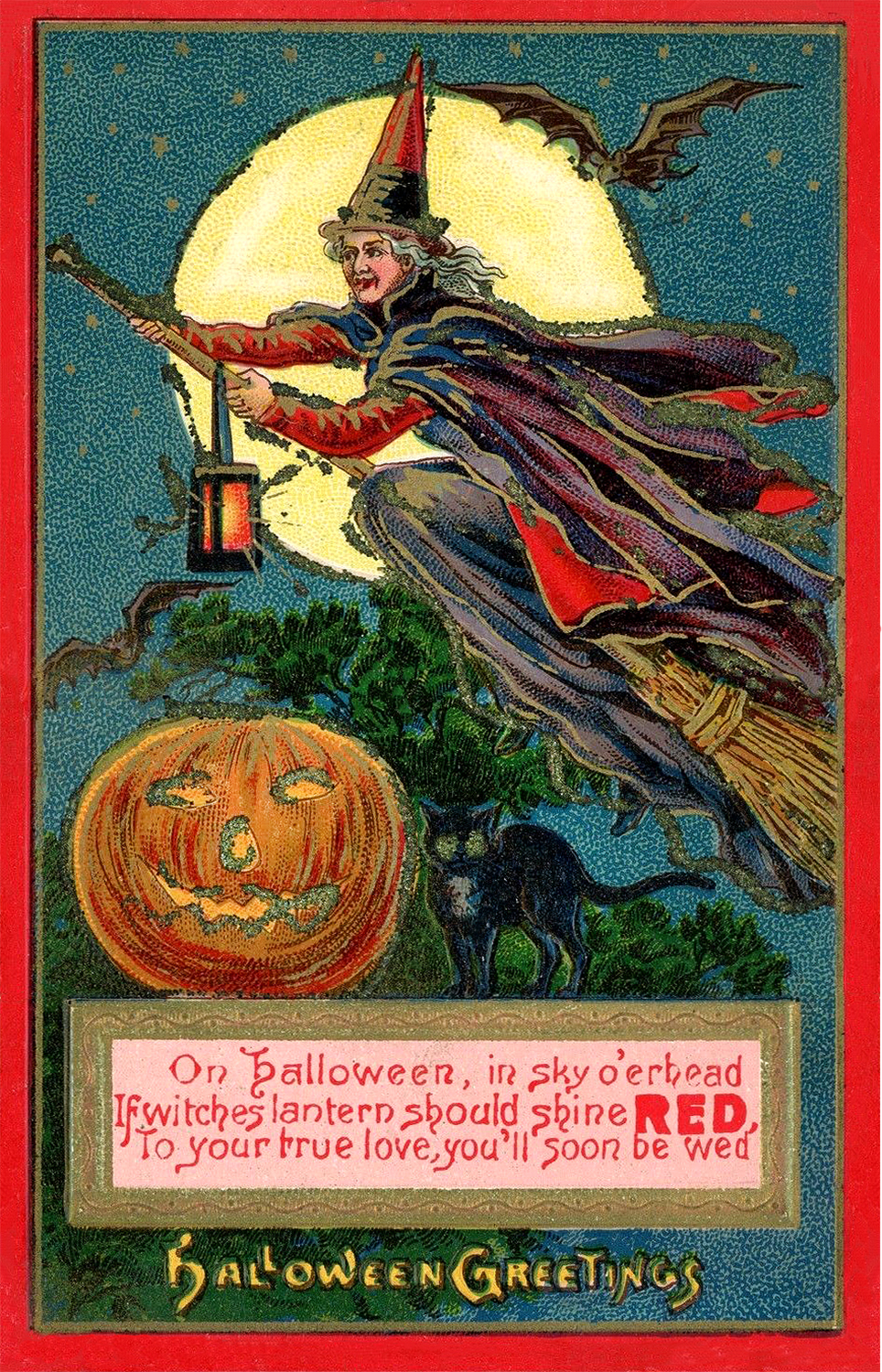This vintage or antique-style Halloween greeting card features a highly stylized illustration of a witch riding a broomstick. The witch, with her flowing white hair, dons a black hat with a red top, a purple and blue cape, and red sleeves. A large yellow moon forms the backdrop, illuminating her figure, while a black bat flies beside her. Below, a grand green tree stretches out beneath the moonlit sky, and a jack-o'-lantern with a classic carved face peeks over the treetop. Perched near the jack-o'-lantern is a black cat with piercing green eyes, gazing directly at the viewer. 

At the bottom of the card, a box with a brown border and red background contains the message in red text: "On Halloween, in sky or ahead, if witch's lantern should shine red, to your true love you'll soon be wed." Beneath this, "Halloween Greetings" is embossed in gold. The entire artwork is composed of meticulously painted small dots, giving it a unique textured appearance. The scene is set against a night sky dotted with faint stars, enhancing the mystical and vintage vibe of the artwork.